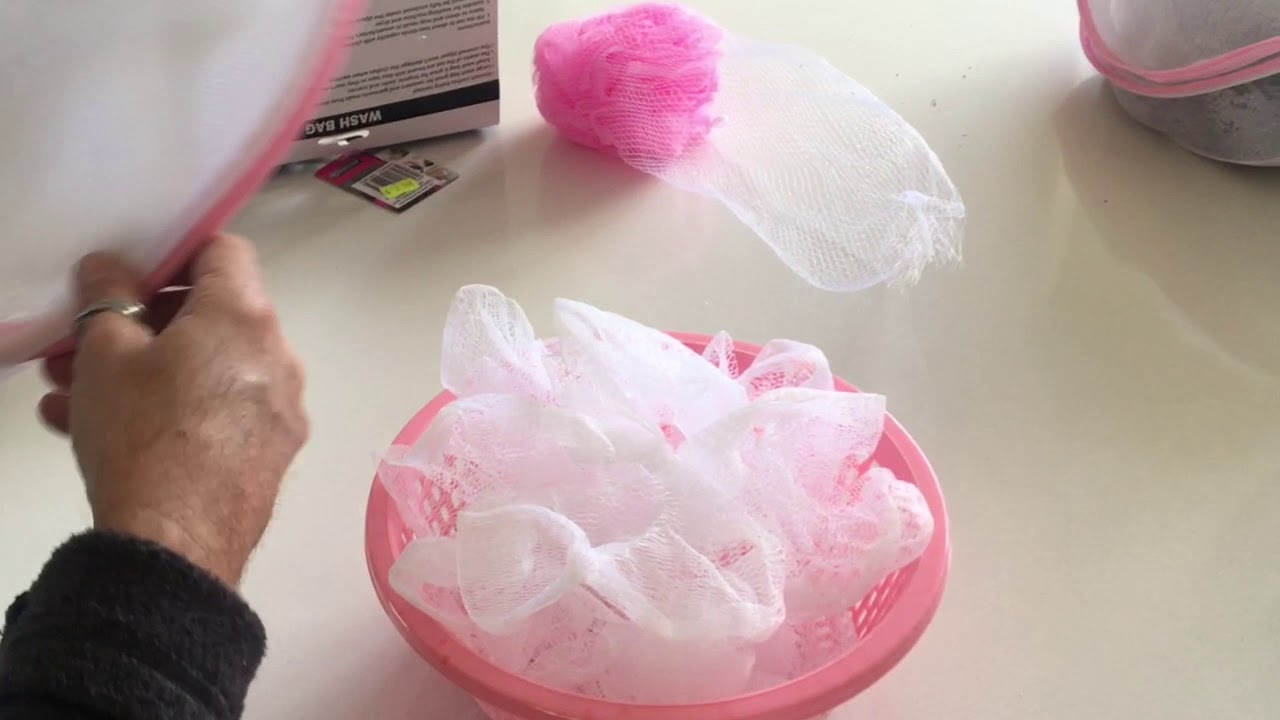This photograph features a central pink colander with holes, presumably resting on a white countertop. Inside the colander, there are several small white mesh bags and some tissues. A bright pink loofah, encased in one of these bags, stands out prominently. To the top right, a different mesh bag with pink piping is visible. In the foreground, a man's hand, adorned with a silver thumb ring and emerging from a grey sleeve, is holding a white object outlined in pink. This object is a wash bag, as indicated by nearby packaging with black and white lettering and a yellow price tag. The overall scene showcases a pink-themed collection, with a pink dish scrubber, a pink wash bag, and pink detailing on other items, indicative of someone's fondness for the color.